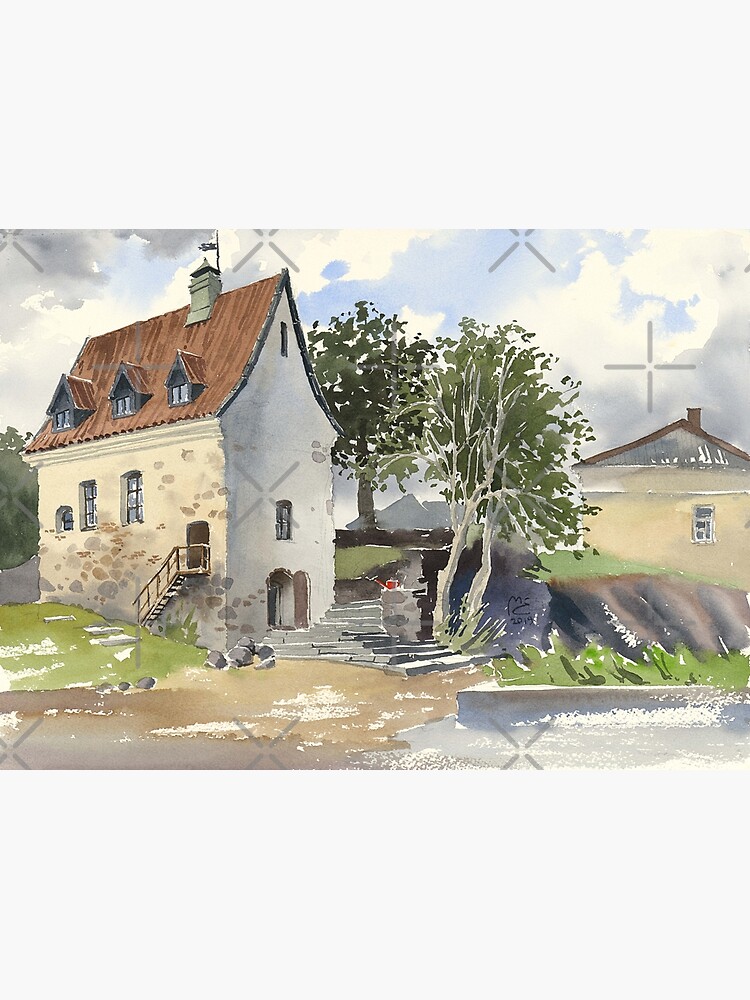The image is a rectangular painting with a thick pale blue border at the top and bottom, giving it a distinctive frame. The painting itself is also rectangular, but oriented so that the top and bottom sides are longer than the left and right sides. Across the painting are semi-transparent watermarks in the form of X's and plus signs, indicating its commercial nature and the need for purchase to remove these marks.

The scene depicts a serene beachside setting with a few buildings. Prominently featured is a two-storied white house on the left side, constructed with a mix of stone and partially worn plaster that reveals the stones underneath. This house has brown dormer windows and a roof, adding rustic charm. Stone steps lead from the beach to the first-floor door of the house, while another set leads up to a grassy area, emphasizing the elevation change from the beach to the residence.

In the middle of the image, a tree stands near the stone steps, providing a touch of nature amidst the built structures. To the right, there is another building partially visible, flanked by another tree. The bottom portion of the painting transitions from a sandy beach on the lower left, which turns into a brown path, to a body of water on the lower right, indicating the proximity to the ocean. The blending colors and seeping effect in the painting suggest it is watercolor, adding a gentle yet vivid touch to the coastal scene.